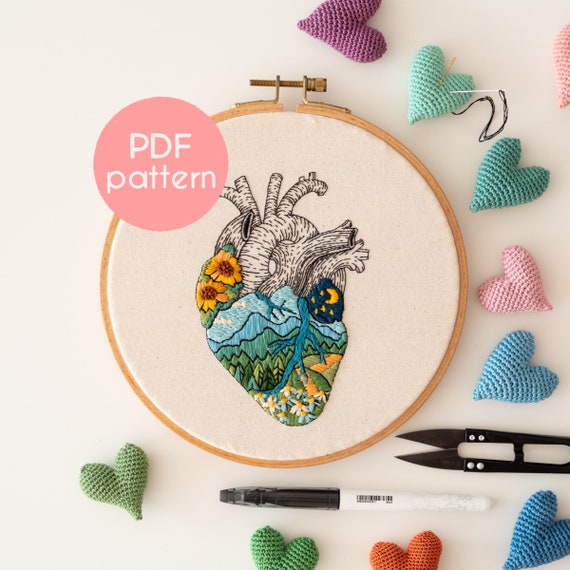This detailed photo features an embroidery art piece showcasing a meticulously crafted anatomical heart within an embroidery hoop. The heart is adorned with diverse and vivid patterns: the top part intricately displays veins and vessels, and the bottom part is richly embroidered with a yellow crescent moon and stars on a dark blue sky. Proceeding downward, blue mountains and green trees transition into a field of white daisies with yellow centers. To the top left of the heart, two sunflowers with yellow petals and brown centers are depicted with green leaves. Encircling the top left corner of the heart, a pink circular label reads "PDF pattern" in white text.

Surrounding the embroidery hoop on a white tabletop are a variety of 3D crocheted hearts in vibrant colors including purple, blue, turquoise, pink, green, and orange. Additional crafting tools such as a black Sharpie marker, fabric shears, and a needle with thread inserted into a seafoam-colored crocheted heart are also present in the composition. The harmonious blend of detailed embroidered elements and colorful crocheted accents creates a vivid and artistic representation.